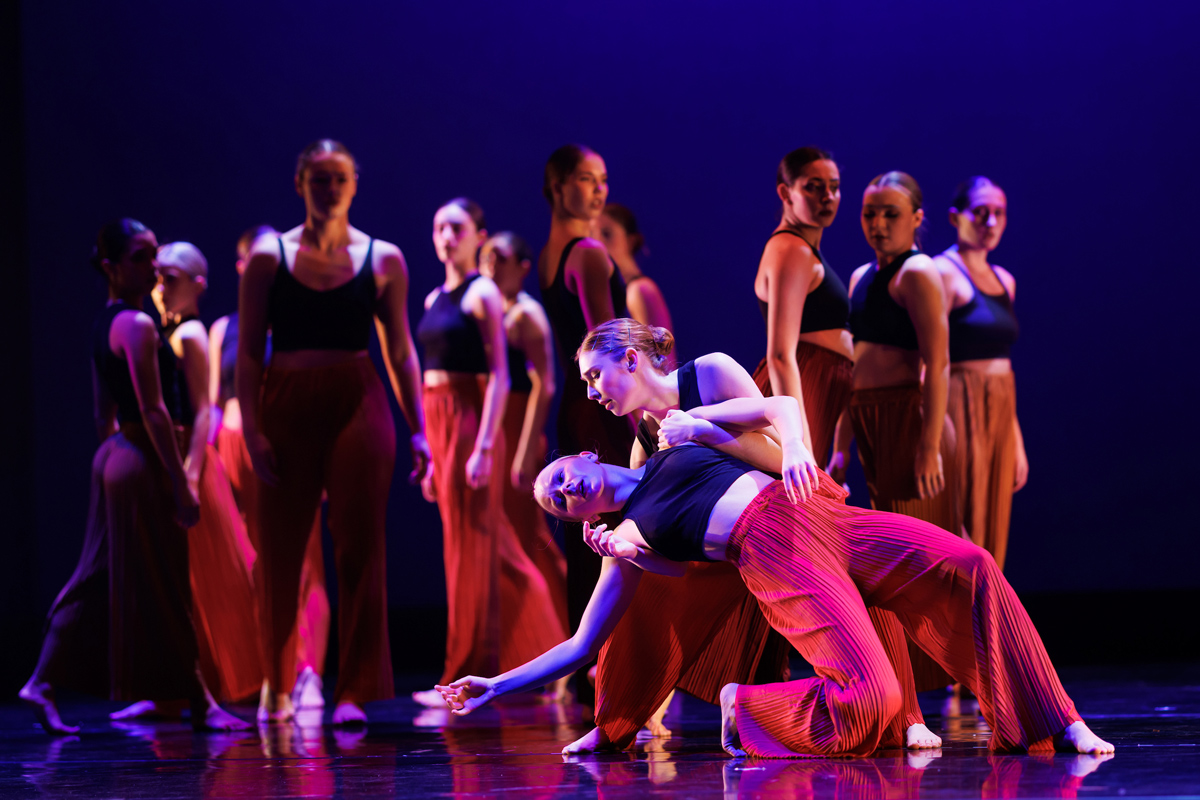This photograph captures a dramatic moment in a modern dance performance featuring an ensemble of about 15 female dancers. The stage is spotlighted, with a dark blue backdrop creating a striking contrast. The dancers are attired in dark sports bra-like tops, some with spaghetti straps, paired with filmy, pleated pants made of a light, somewhat see-through fabric in varying shades of red and brown. In the forefront, two dancers command attention: one is leaning dramatically backward while the other appears to be supporting her from behind, kneeling. This intense pose draws the gaze of the other dancers, who stand erect in the background, seemingly paused and observing the central action with concern or focus, as though awaiting their cue to rejoin the performance. Their bare feet add to the grounded, earthy aesthetic of the scene, which vividly portrays the emotive power and physicality of modern dance.